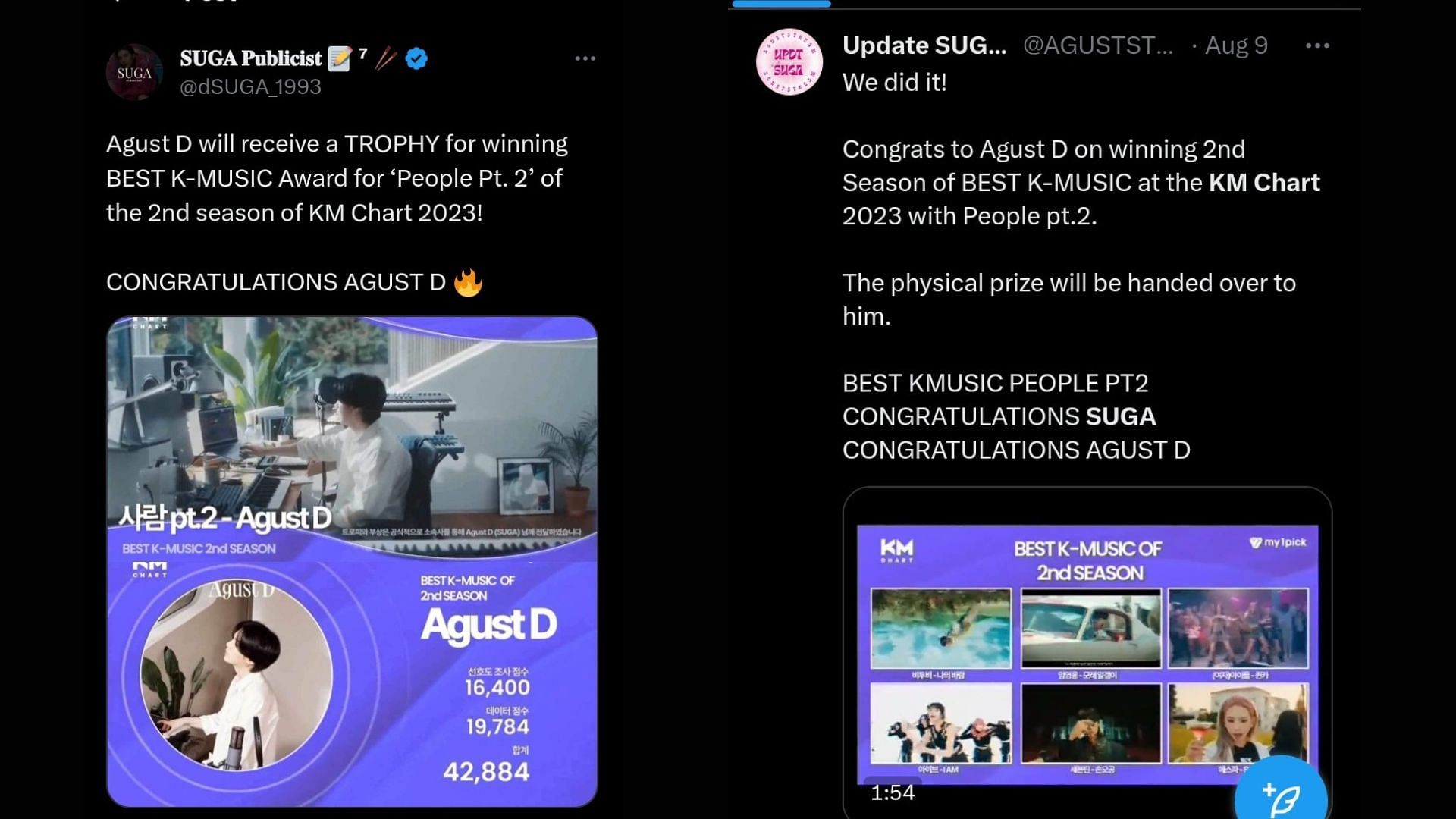This is a detailed left-to-right horizontal image, showcasing a social media post, likely from Twitter, which can be viewed on both smart devices and computers. The image features a sleek, black background with a small blue line centrally located. The background has no texture and appears as a smooth, one-dimensional, solid black color.

On the left side of the image, there is a circular profile picture accompanied by text in white that reads "Suga Publicist." Next to it are several icons and the handle "@Suga_1993." The post mentions: "August D will receive a trophy for winning Best K Music Award for 'People 0.2' of the second season of KM Chart 2023. Congratulations, August D! 🔥"

Below this text is an image, presumably of the artist August D, highlighting his accolades.

Following this, there is another section with a different profile picture from "Update S-U-G," and the handle "@AugustST." The post says: "August the 9th. We did it! Congrats to August D on winning the second season of Best K Music at the KM Chart 2023 with 'People Part 2.' The physical prize will be handed over to him. Best K Music People Part 2. Congratulations, Suga. Congratulations, August D."

In the final part of the image, there is an outlined box in purple that reads "Best K Music of the second season." Inside this box are three pictures on the top row and three pictures on the bottom row, likely depicting either moments from the event, the artist, or other celebratory images.